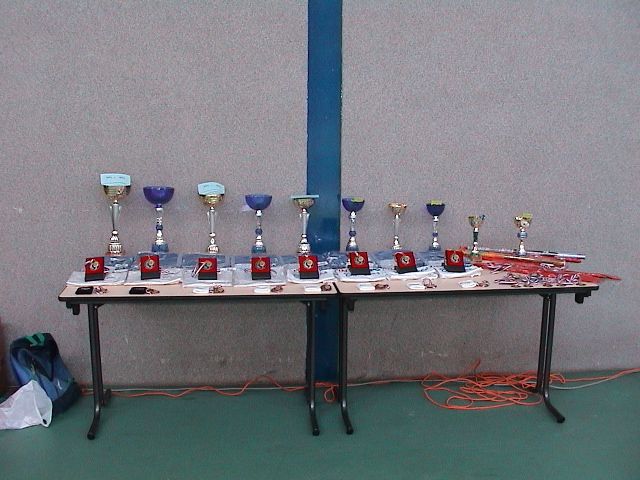The image depicts an outdoor setting with a green, possibly cement, floor and a grayish-pink wall that features a blue divider. Against this wall, there are two rectangular tables with metal legs, placed side by side. An orange extension cord runs along the bottom of the wall and is coiled in a pile on the right side of the image. On top of these tables is a well-organized display of trophies, medals, and pins. The trophies, which vary in size with some exceptions, decrease in height from left to right and include both silver and colored cups, such as a clear blue glass and a purple cup. Each trophy has a placard in front of it, and preceding the placards are other small objects, possibly trinkets or creations. Additionally, a blue backpack with a green tag and a white plastic bag are situated near the coiled extension cord.